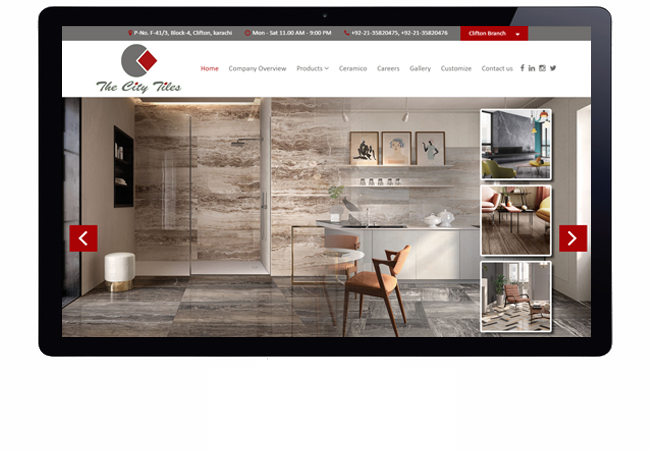This screenshot captures the homepage of a website specializing in tile sales, prominently branded as "City Tiles" in the top left corner. The main feature of the page is a large, high-resolution image showcasing a luxurious room, possibly an office or sitting room, adorned with elegant marble tiles on both the floor and walls. On the right-hand side, there are three vertically stacked image thumbnails, allowing users to click and view additional visuals. Furthermore, navigational arrows on both the left and right sides of the main image facilitate easy scrolling through a gallery of images.

In the upper navigation bar, directly to the right of the "City Tiles" logo, are several menu options including "Home" (currently highlighted in red), "Company Overview," "Products," "Ceramics," "Careers," "Gallery," "Customize," "Contact Us," and icons for social media platforms like Facebook, LinkedIn, Instagram, and Twitter. These icons suggest that the company maintains an active presence on these networks, providing additional avenues for customer engagement and brand promotion.